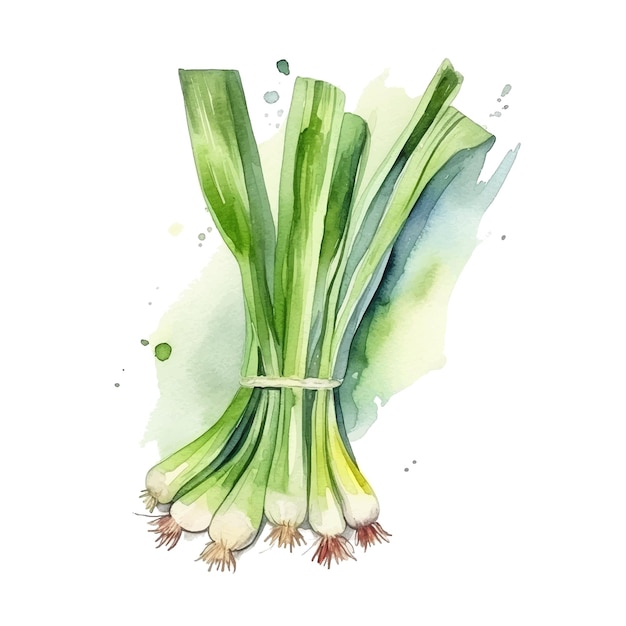This vertical, cartoonish watercolor painting depicts a bunch of six scallions, tied together with a white rubber band. The scallions feature bulbous white bottoms with brown, stringy roots extending from them, transitioning into broad green leaves as they ascend. One scallion in the middle is distinguished by a white stripe running its length. The background consists of a splotchy mix of green, dark blue, and yellow hues, enhancing the vibrant, animated aesthetic of the illustration.